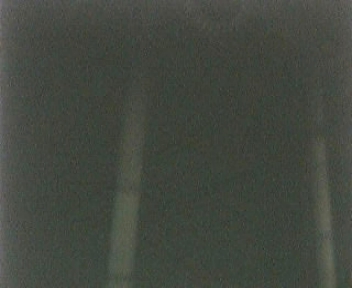This image is a very dark and blurry photograph with a gray and black background, possibly taken at night or in low-light conditions. The picture appears to have low quality, with visible pixelation and little gray spots scattered throughout. There are two vertical lines or poles resembling bamboo sticks. One is positioned on the left side, extending from the bottom to nearly the top, while the other is slightly towards the center but more to the right, also extending vertically. An unclear arc is faintly visible above, adding to the image's overall distorted and unclear nature. The photograph seems to be in black and white, enhancing its void and darkness.